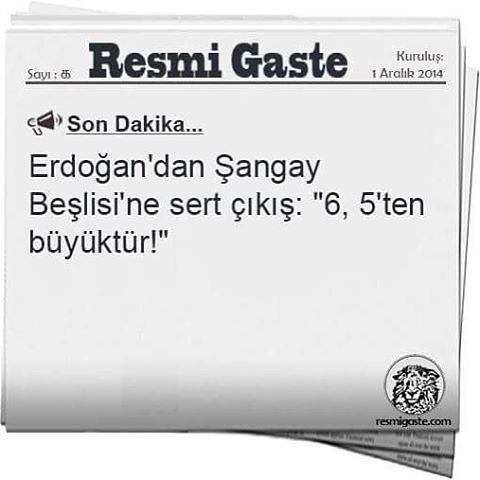The image is a graphic representation of a Turkish news notification from 2014, showing a series of stacked white folders. The main visible folder features bold black text at the top that reads "RESMIGASTE," followed by a megaphone icon and the phrase "SONDAKIKA." Below this, the text continues in Turkish, mentioning "Erdogan." The notification includes various headings such as "SAYI" and "KURLUS," and details like "ARALIK 2014." There is also a black and white logo of a lion's face at the bottom right, and the website "resmigate.com" is displayed. The design suggests that there are multiple similar notifications beneath the top one, indicated by the visible corners and edges.